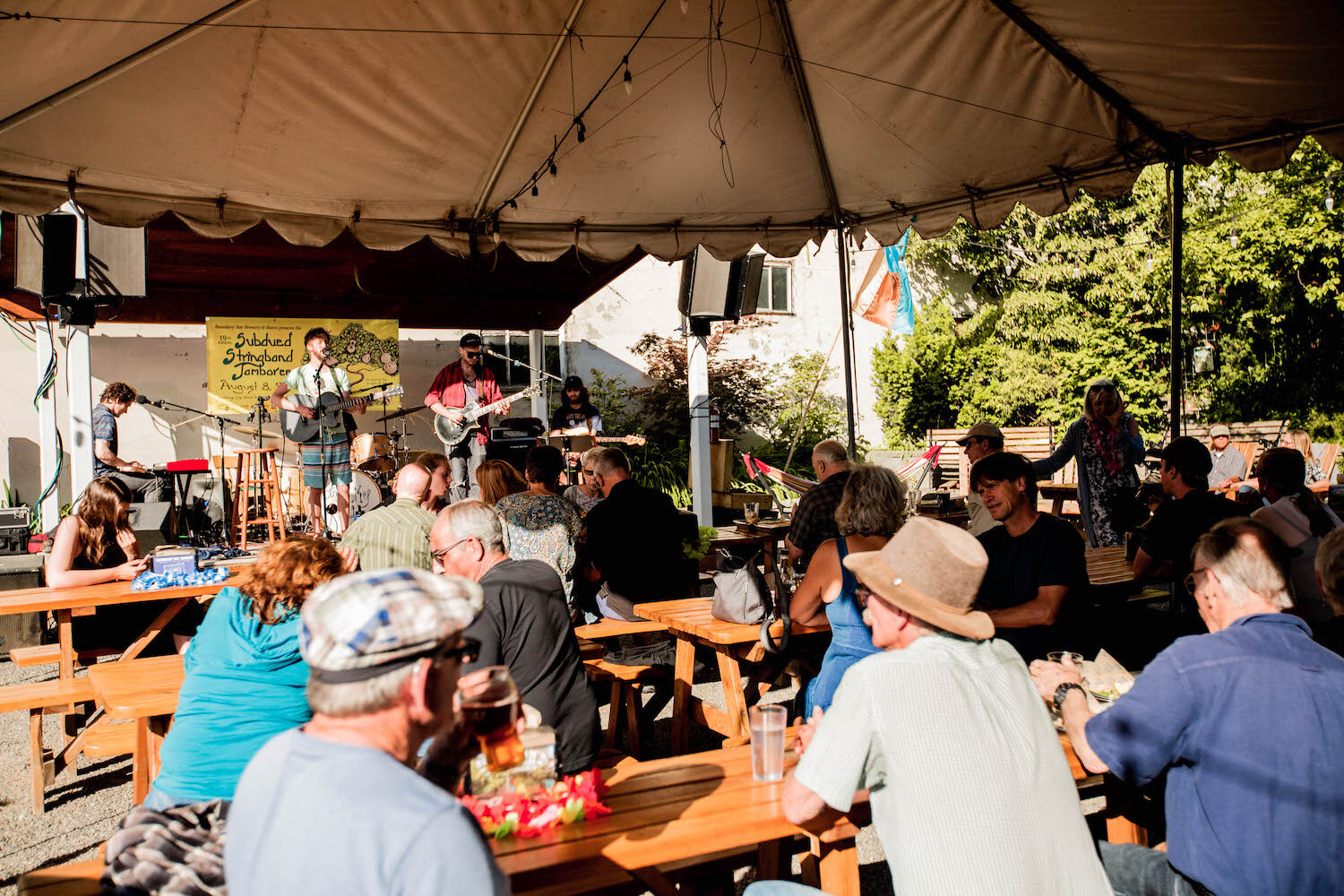In this outdoor scene, a bustling festival unfolds beneath a large tan canopy tent that shelters rows of wooden picnic tables. An older, middle-aged crowd is seated with their backs to the camera, many chatting and sipping on drinks as they watch a live band perform on stage. The stage itself is covered by a wooden canopy and decorated with a yellow banner with green letters that read "Subdued String Band Jamboree." 

Onstage, a man with an acoustic guitar sings into a microphone, while to his right, another guitarist in a red shirt plays a black electric guitar. Seated farther right, a bass player can be seen, and to the left, a man plays the keyboard. The scene is anchored by white poles, which hold speakers that amplify the band's melodies to the intimate gathering of about 30 people. A sense of community and shared enjoyment permeates this lively, yet cozy festival atmosphere.